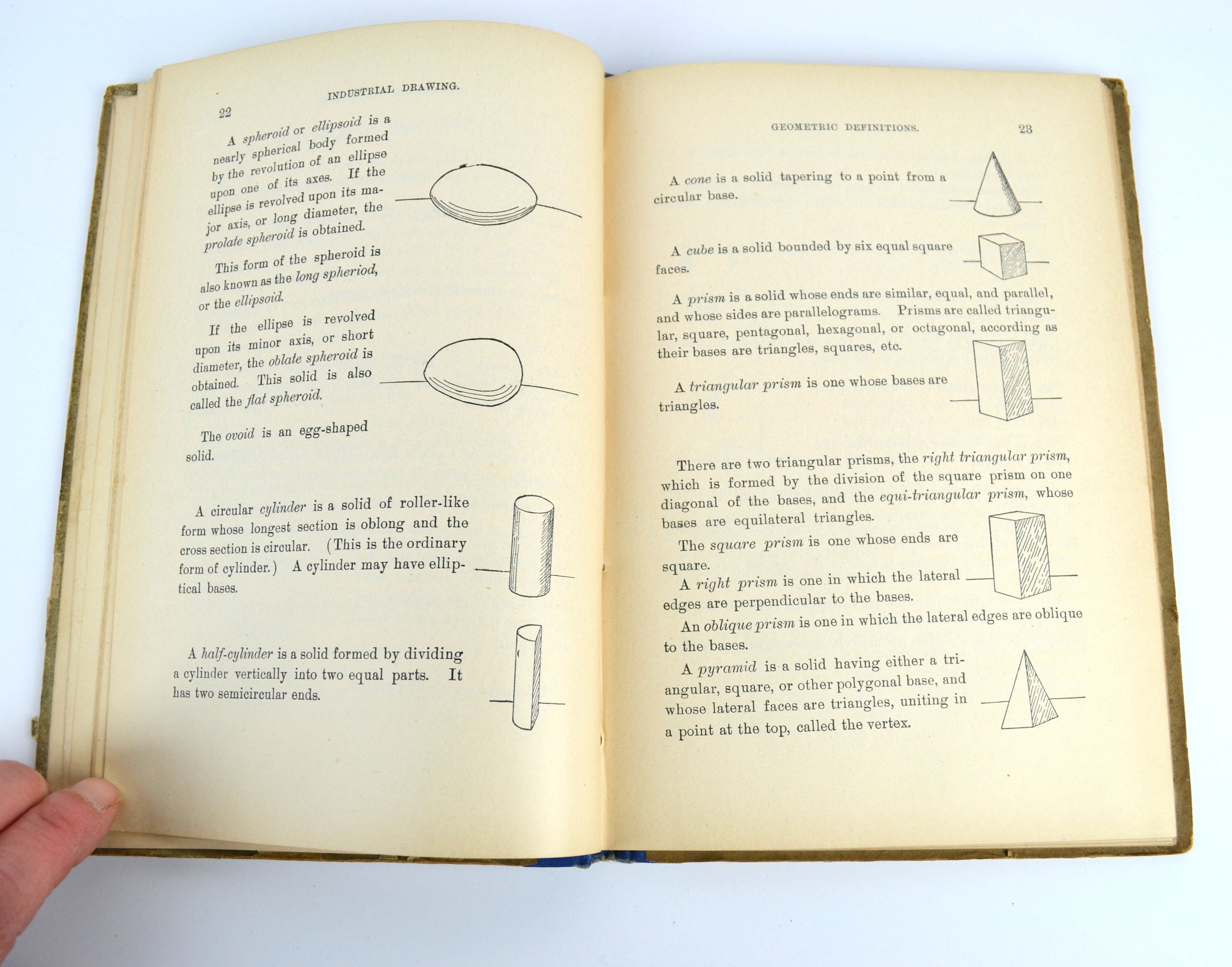The photograph features a large, vintage textbook, its pages distinctly yellowed with age. The book is open to pages 22 and 23, with "Industrial Drawing" heading the left page and "Geometric Definitions" heading the right. Detailed 3D geometric sketches fill both pages: the left page includes illustrations and text about ellipsoids, ellipses, egg shapes, cylinders, and half-cylinders, while the right page features cones, cubes, prisms, triangles, tall blocks, and pyramids. Both pages have numbers at the top corners - 22 on the left and 23 on the right. The book lies on a light-colored table, taking up most of the frame, with a few fingers of a white person's left hand visible in the bottom left corner, touching the book gently.